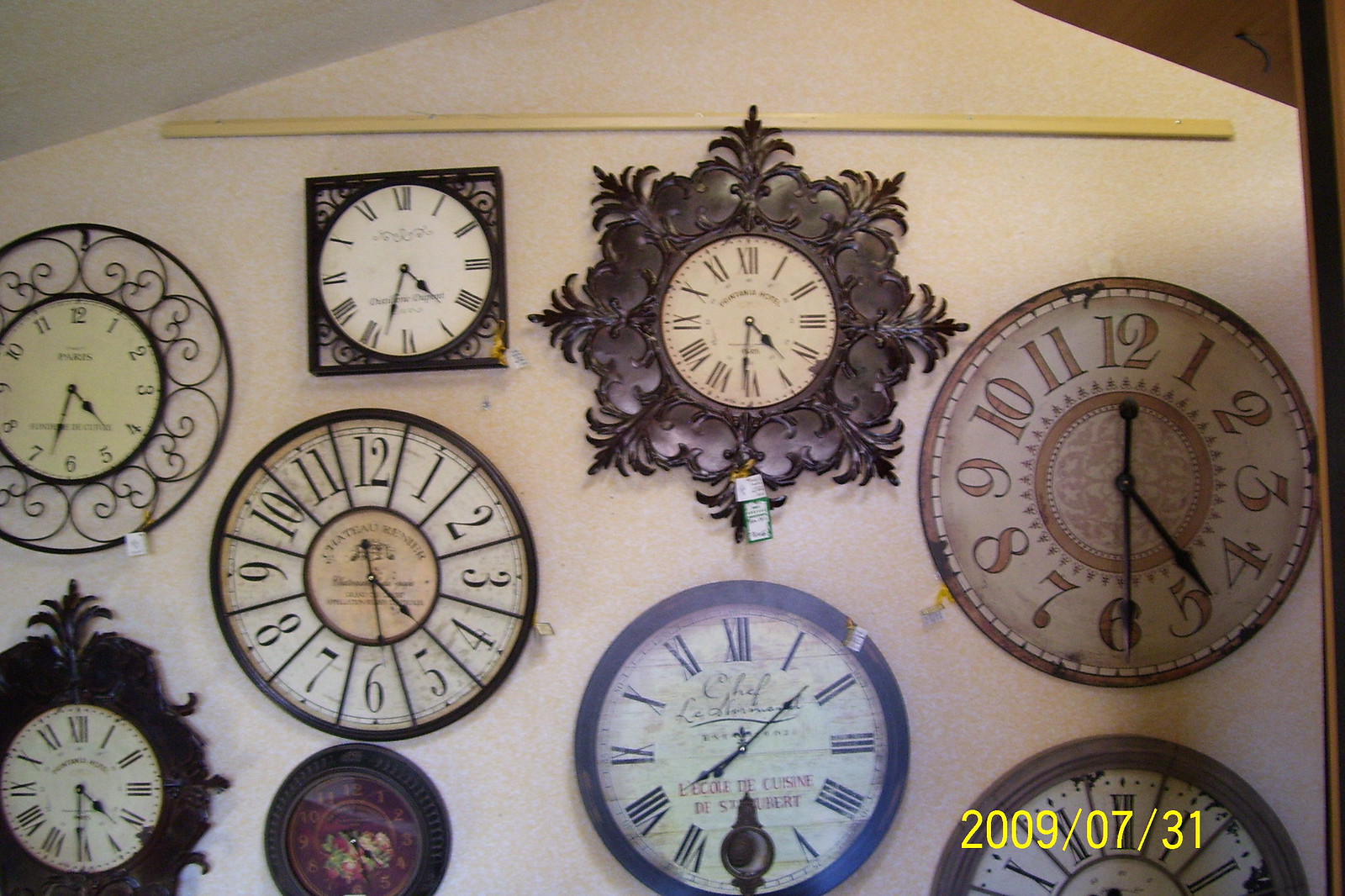The photograph captures a light beige wall with a subtle pattern, possibly tinged with a yellowish hue. The ceiling at the top of the image is angled, accentuated by a horizontal wooden dowel or rod. Nine variously designed and sized wall clocks adorn the wall, mostly round with a couple featuring ornate square or flowery borders. One prominent clock near the top center has a black flowery design encircling its face, while another on the right side is characterized by brown numbers and a central sun-like motif. Another noteworthy clock in the lower right corner boasts a fancy black fleur-de-lis design and Roman numerals, complete with a date stamp at the bottom reading "2009-07-31." Most clocks appear to show the same time, around 4:30, highlighting their synchronized nature.